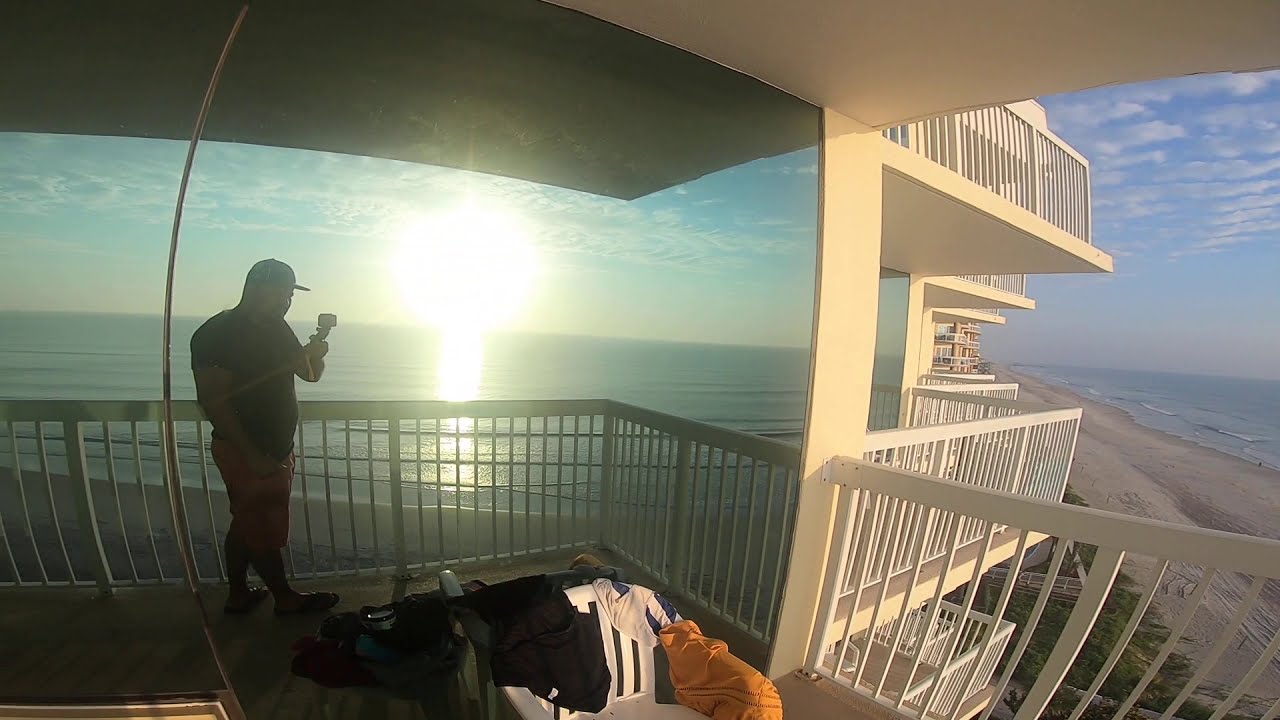In this detailed image, we see a scene taken from the balcony of a beachside apartment or condominium complex. The vantage point is slightly diagonal, showcasing both the complex and the beach on the far right. The sun, positioned low in the sky and bright, illuminates the scene, reflecting brilliantly off the ocean water. This reflection is mirrored in the glass window of the building, creating a striking visual effect. The sky above is a vibrant blue, dotted with numerous clouds.

On the balcony, cluttered with various items, there's a white plastic chair draped with clothes in black, white, and orange. The building's exterior is a light cream or very pale yellow, complemented by white-painted balconies, suggesting a well-maintained complex. In the foreground, a man in a black shirt, shorts, and a baseball cap is observed, possibly taking a photograph, with his hand in his pocket. Farther off to the right, the sandy beach and breaking waves are visible, adding to the serene coastal ambiance. Other similar balconies, probably part of the same complex, can be seen extending to the right, pointing to a larger, multi-unit living facility.